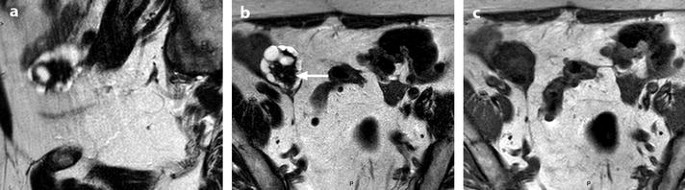This image presents a detailed triptych of black and white X-ray or MRI scans, labeled consecutively with lowercase letters 'a', 'b', and 'c' in the top left corners of the respective sub-images. Each sub-image reveals various intricate shapes in shades of black, gray, and white, signifying different densities and structures within the scanned area. The focal point across these images appears to be a nodule located towards the top left section of each scan. In image 'a', the nodule features a black core with an internal white area surrounded by a somewhat blurry coating. Progressing to image 'b', an arrow points to the now more defined nodule, which retains its black core and peripheral white blobs, though it appears somewhat rotated. By image 'c', the nodule is depicted entirely in dark shades, and the internal light areas have disappeared, indicating a change in composition or state. These images, likely used in a scientific or medical context, compare the progression or variance of this nodule, potentially illustrating stages of an abnormal cell formation or other significant biological phenomena.